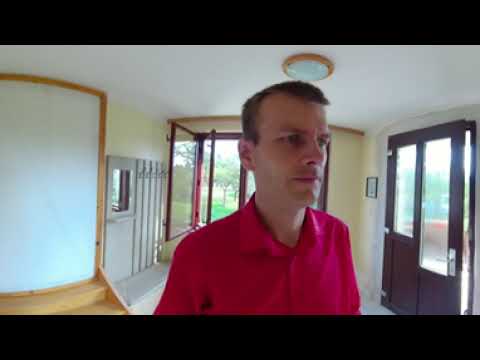The photograph captures a man in his 30s with short brown hair, slightly receding at the hairline, dressed in a button-down, long-sleeved red shirt. He stands at the center of a room, which appears to be part of a house, bathed in daylight streaming through the windows. The man is looking slightly to the right side of the image, with a neutral expression on his face. The room features a round ceiling light with a gold ring and a hazy white lens, adding a calm ambiance. To the right, there is an open doorway leading to another room, while to the left, a staircase can be faintly seen. A pair of double doors, with one door open, stands prominently behind him. The windows reveal a view of trees outside, emphasizing the daytime setting. Near the back left corner, an open window is positioned above a bench, with coat hooks mounted on the wall, indicating a space to store personal items. The photograph is framed with black lines at the top and bottom, and there is no identifying text or information about the exact location. The color scheme includes hints of white, brown, red, green, tan, and gold, creating a warm and homely atmosphere.